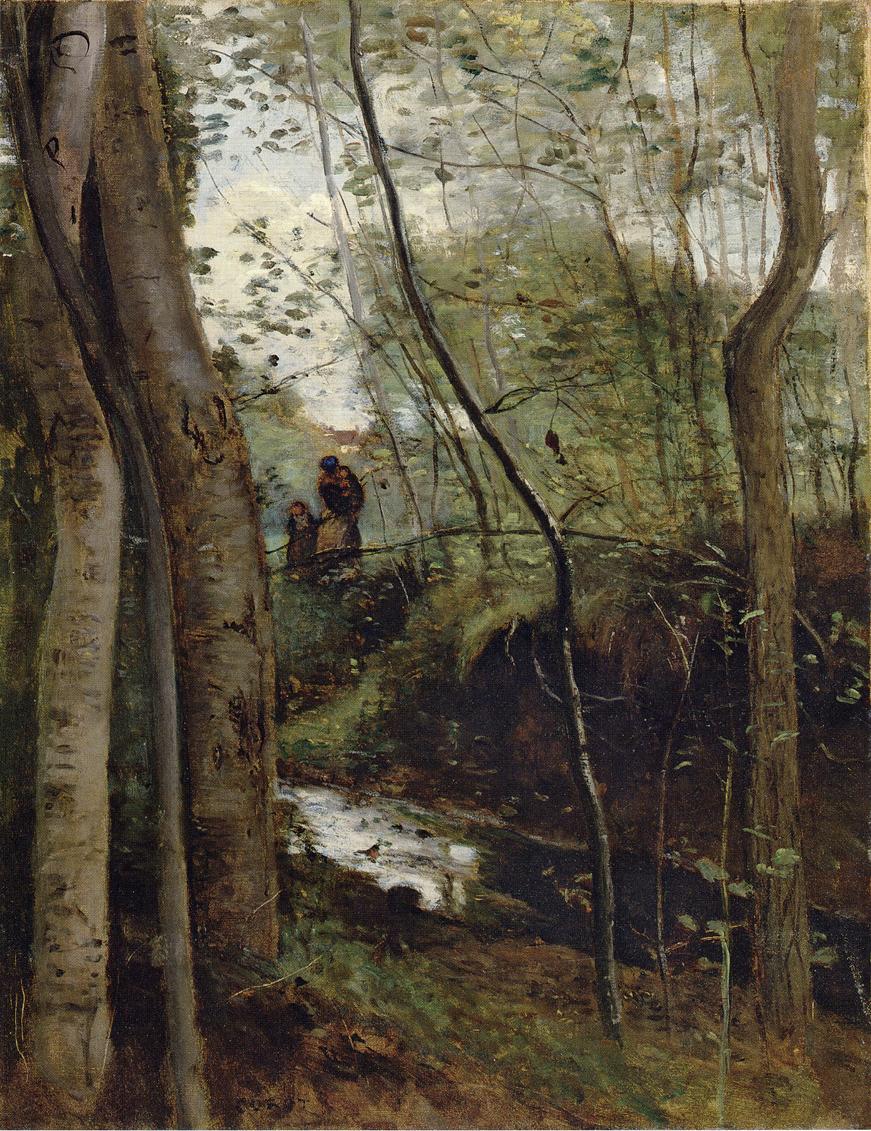This highly detailed and realistic painting depicts a serene scene in a country forest. Dominated by a wooded area with a meandering creek, the foreground showcases three prominent, crooked trees with visible markings and an undergrowth of small plants with green leaves. At the bottom left, the trees reach upwards, and a realistic depiction of tree branches intersperses the scene. The background extends into lush green hills and a canopy of tall trees, with glimpses of a pale blue sky dotted with puffy white clouds indicating a spring or summer setting.

Central to the composition, spanning the creek, are two adult figures, one appearing older and dressed in a robe with a blue cap, likely holding a child. Beside them are three smaller figures, possibly children, dressed in what appears to be historical attire. The smaller children, with one potentially being a boy and two possibly little girls in dresses and hats, add a nostalgic, antique quality to the scene. Their presence, along with the sky's reflection in the creek, enriches the painting's depth and historical allure, further anchoring the viewer in the tranquil, timeless forest landscape.